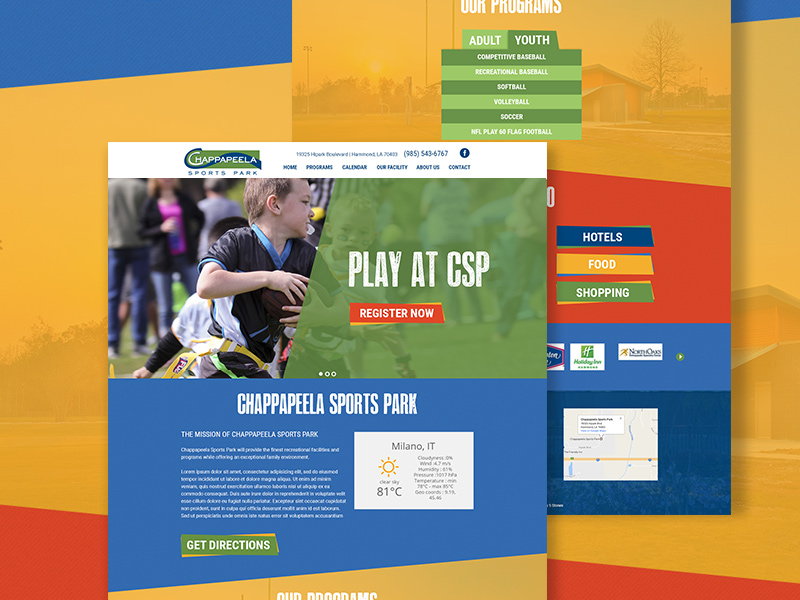**Detailed Caption:**

The screenshot depicts a vibrant and colorful background featuring modern art-inspired splashes of bright blue, golden yellow, and red hues. Dominating the foreground is a central screen showcasing information about Chappapila Sports Park. Across the top of this screen, the header includes the text "Chappapila Sports Park" along with a contact number, "985-543-6767," and a link to their Facebook page.

Beneath the header, a navigation bar lists several tabs: Home, Programs, Calendar, Our Facility, About Us, and Contact. The center of the screen displays an image of a young child dressed in a sports uniform, actively engaged in a sports activity. Adjacent to this image, a green background shape contains the prompt "Play at CSP, Register Now."

Below the child's photograph, a blue shape reiterates "Chappapila Sports Park," along with a brief mission statement, which is unfortunately too small to decipher. Further down, there is a "Get Directions" link.

To the right, a white rectangle labeled "Milano, Italy" includes an icon of the sun and indicates the temperature is a scorching "81 degrees centigrade," with additional, smaller text beside it.

The lower section of the screen presents a green and lime green box titled "Our Programs," listing different sports opportunities: Adult, Youth, Competitive Baseball, Recreational Baseball, Softball, Volleyball, Soccer, and Flag Football.

Beneath this section are buttons for Hotels, Food, and Shopping, leading to an extensive listing of nearby hotels and a map for reference.